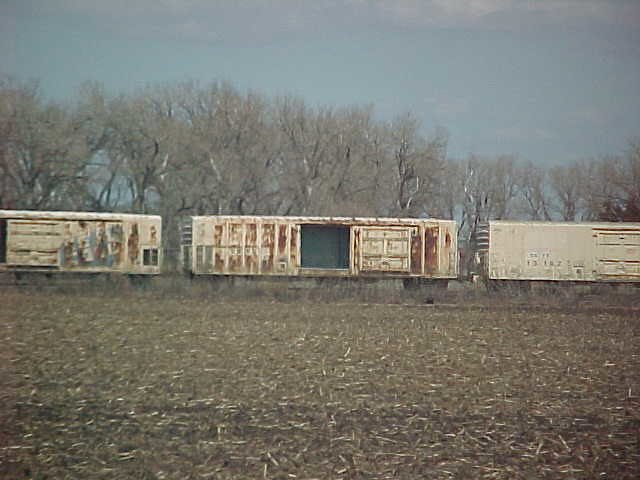In this grainy, faded photograph, three large, cream-colored train cars, heavily marked with brownish-red rust, stand in a desolate farmer's field. The central train car has its door wide open, revealing an empty, gray interior, while the other two are closed but similarly rusted. The foreground is littered with dead straw or corn husks scattered along the brown dirt, indicative of a recently harvested field. Tall trees, bare of leaves, form a stark backdrop, their branches reaching skyward against the light blue daytime sky. The scene, likely captured during a dry and possibly cold season, evokes a sense of abandonment and decay.